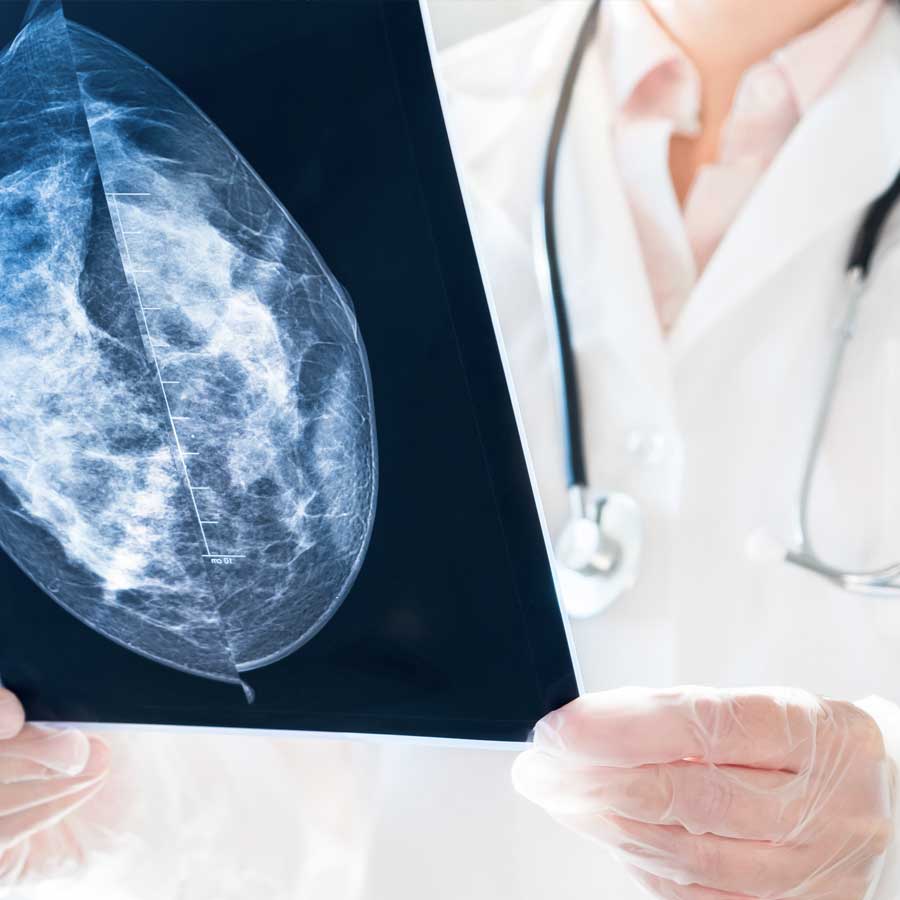The image depicts a professional medical setting focused on a doctor or nurse, identifiable by a white medical coat over a pink (salmon-colored) shirt. From the neck down, the individual is dressed with clear white medical gloves and has a black stethoscope with silver details hanging around their neck. The photograph is a close-up shot, showing the person's hands and torso, stopping just before the neck.

In their gloved hands, the medical professional is holding an x-ray that appears to show a brain or skull. The x-ray is predominantly black with greys, blues, and whites forming an image that suggests the internal structure of the skull or brain. The scan seems to be trimmed in black and might appear split, though rejoined without any visible gaps. This detailed scene encapsulates a moment of clinical examination or diagnosis, emphasizing the precision and care inherent in medical practice.